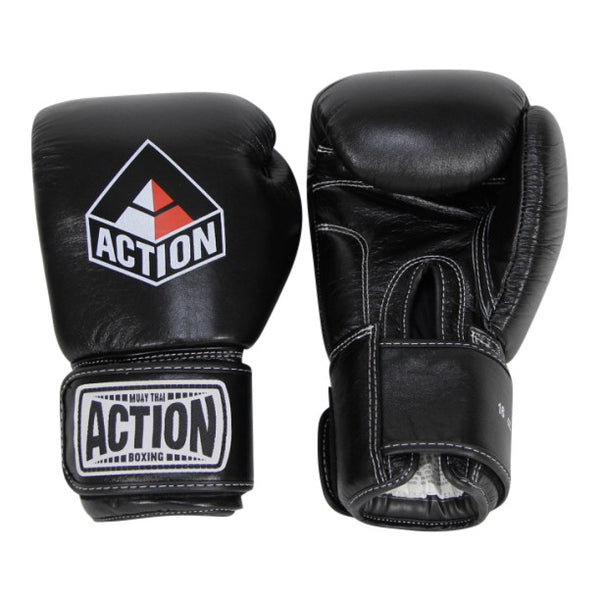This image features a photograph of a pair of black boxing gloves against a white background. The left glove is positioned to show the back of the hand, showcasing a logo that reads "ACTION" beneath a pyramid-shaped icon, all in white. The wrist strap also bears the text "ACTION BOXING" with contrasting black and white stitching. The right glove is oriented to reveal the palm, highlighting the white interior and the detailed white stitching that runs along its black exterior. The gloves are crafted with a clean, high-quality black leather finish, making the image suitable for a product listing, possibly for online sale.